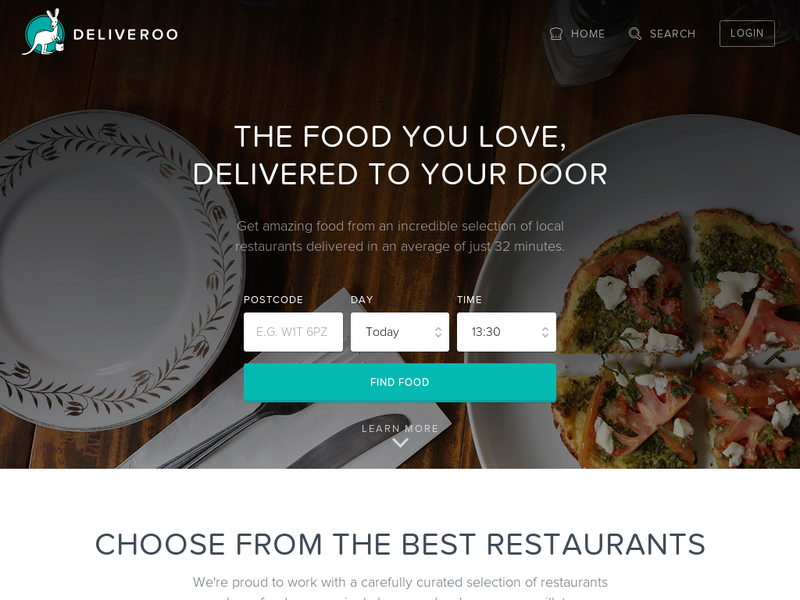This is an advertisement for Deliveroo, prominently displaying their logo in the upper left-hand corner. The logo features a kangaroo inside an aqua circle holding a bucket, emphasizing their food delivery service. 

On the opposite side of the page, options for "Home," "Search," and "Login" are clearly visible. The central tagline reads: "The food you love, delivered to your door." The advertisement highlights that users can receive amazing food from a curated selection of local restaurants, delivered in an average of just 32 minutes.

Users are prompted to enter their postcode, select today's date, and specify a delivery time of 1:30 PM. Below this form, an aqua-colored button labeled "Find Food" is prominently displayed, with a "Learn More" link and a downward arrow beneath it. 

The accompanying text encourages users to "Choose from the best restaurants," stating that Deliveroo collaborates with a carefully curated selection of eateries. The background image features a wooden table set with a plate, fork, and knife on a napkin. A larger plate displaying a delicious Margherita pizza is also part of the visual.